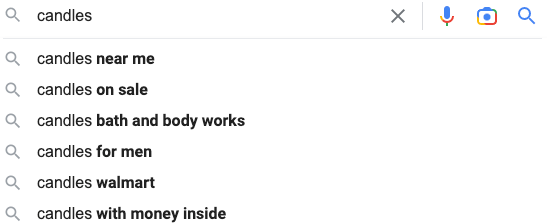This image is a screenshot showcasing a Google search interface. At the top of the screen, a search bar is prominently displayed, containing the typed word "candles" in small, lowercase black font. To the left of the search input is a small magnifying glass icon, denoting the search function, while to the right, an "X" icon allows users to clear the search term if needed. 

Adjacent to the "X" icon, there are three additional smaller icons offering various search functionalities: a microphone for voice search, a camera for visual search, and another magnifying glass which initiates the search when clicked.

Below the search bar, Google provides seven suggested search queries related to the term "candles," each accompanied by a small magnifying glass icon for easy selection. The suggestions include "candles near me," "candles on sale," "candles, bath and body works," "candles for men," "candles, Walmart," and "candles with money inside." Users can click on any of these options to refine their search based on specific interests or needs.